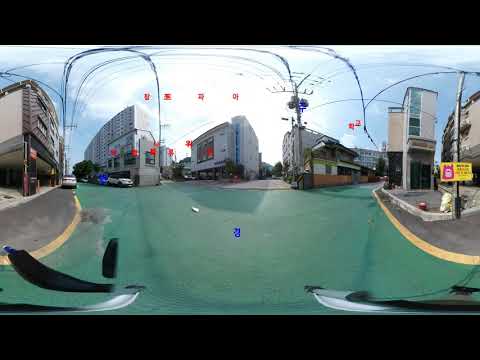This image is a panoramic view of a city intersection marked by a distinctly green road that transitions into the typical light gray asphalt further down. The intersection features bright yellow stripes and unmarked lanes, with a yellow-painted curve leading to a slightly elevated, dark-colored concrete pathway. Overhead, telephone wires crisscross above the multi-storied rectangular buildings in white, tan, and gray hues. The panoramic nature of the photograph creates some distortion, suggesting multiple streets converge in complex angles around the central vantage point. Despite the daytime setting with patches of blue sky and partial cloud cover, the streets are notably empty. Chinese characters appear in a clear banner format across the scene, adding a unique cultural touch. The visual might evoke a resemblance to places like Atlantic City due to the mix of urban structures and open skies.